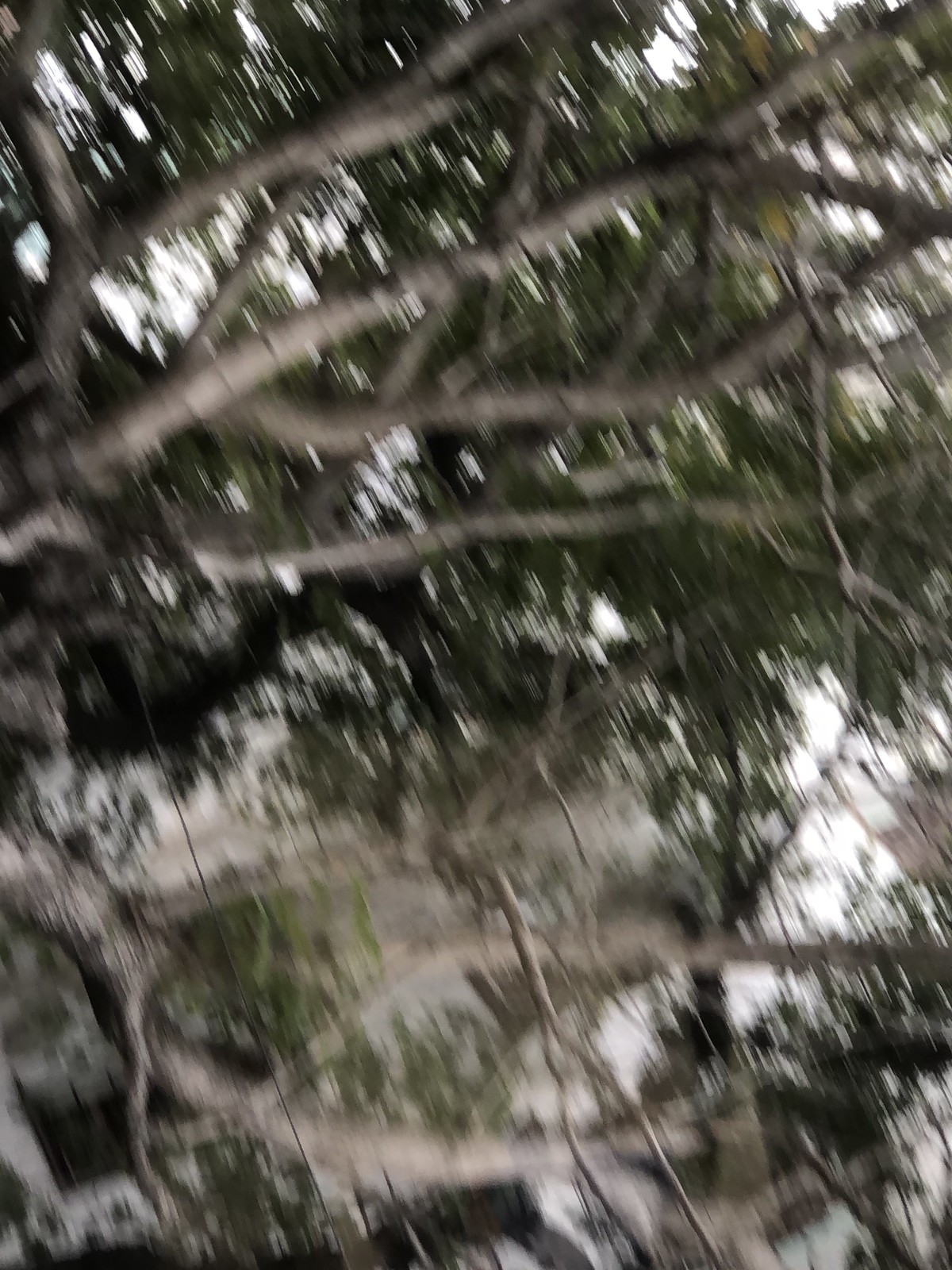This outdoor photograph captures a ground-up perspective through the branches of a tree, resulting in a slightly blurry and dimly lit image. The tree branches, adorned with smooth yet occasionally rough, light gray bark, stretch upwards and frame the composition. The dark green leaves, though indistinct due to the blurriness, form a dense canopy. Punctuating this leafy network are glimpses of a pale, almost white sky, most noticeably visible in the bottom right and top left corners of the photograph. The overall effect is one of a serene, slightly mysterious woodland scene observed from a unique viewpoint.